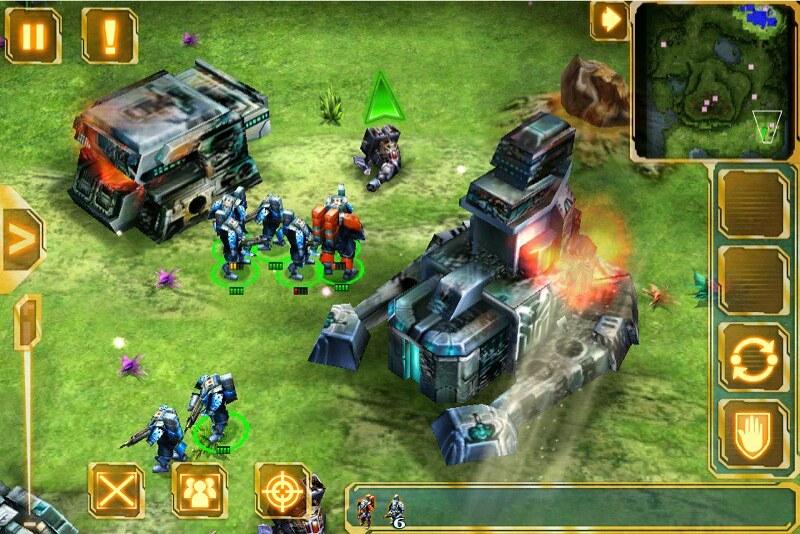The image is a detailed screenshot from a mobile game inspired by Starcraft. In the central part of the screen, there are heavily armored, weapon-bearing alien troops moving around on green grass, each distinctly marked with green circles underneath them for selection. Dominating the middle of the battlefield is a large, mostly gray futuristic structure, with several tier-like sections and an orange light reflecting off its bottom right side.

On the upper left corner of the interface, there are control icons including a pause button and an exclamation point. The bottom left displays various action-related icons: an "X" symbol, a silhouette of three heads, and a bullseye target sight. On the top right is a small square minimap with pink square markers indicating key points within the game. Below this minimap, there are four gold-colored buttons with gray centers; one of these buttons has symbols indicating a badge and a hand in the middle.

In the primary frame, alongside the large structure, multiple robot-like military units are visible, each equipped with various rifles and guns, contributing to the game's military and war theme. The overall color scheme prominently features shades of green and gray, encapsulating the tactical and alien environment of the gameplay.